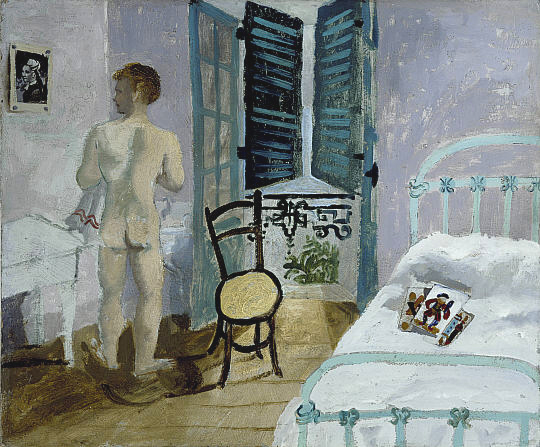The painting depicts a bedroom scene with a man standing nude beside a white basin on the left. His back, painted in shades of gray, stretches from top to bottom, accentuating his red hair. He turns his head towards the left, staring intently at a portrait of a woman against a black background, framed in white, that hangs on a pink, paint-peeling wall. A white and red striped rag dangles from his left side. In front of the man is an open window, flanked by blue shutters, which offers a view of green foliage and a metal wrought wire railing through an open screen door. To the right, a bed with a light green frame and a white comforter lies beneath an open magazine. A brown chair with a light cream seat sits on the ground nearby, complementing the brown streaked floor. The overall style of the painting evokes the brushstrokes and color palette reminiscent of Van Gogh.